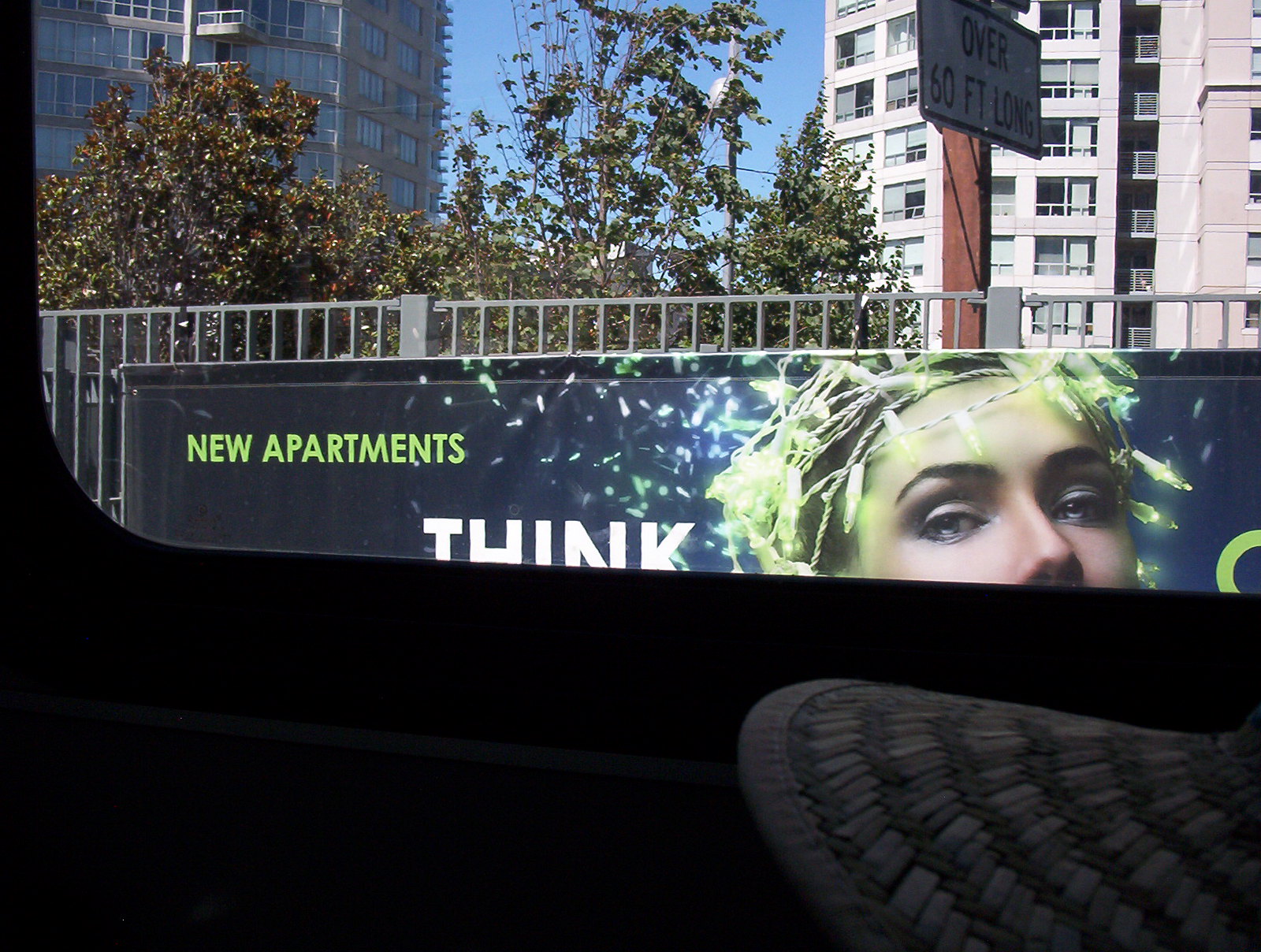This image, taken from the window of a bus, captures an urban cityscape. The foreground inside the bus is dark, providing a stark contrast to the bright scene outside the window, which reveals high-rise apartment buildings with balconies under a clear blue sky. In the background, green trees add a touch of nature to the city environment. Prominently featured is a large mural advertisement for new apartments, depicting a woman's head adorned with Christmas lights, though only the upper portion of her face is visible up to her nose. A red pole-mounted sign states "Over 60 feet long," possibly indicating an upcoming tunnel or bridge, and a silver fence can also be seen. The bottom right corner of the image displays the brim of a wicker hat, suggesting the presence of a person inside the bus.